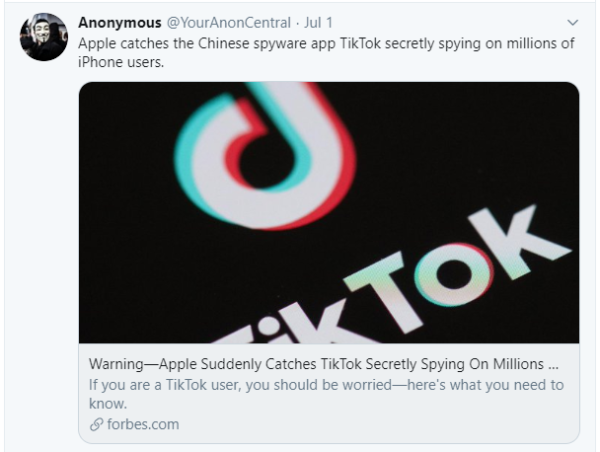A detailed and cleaned-up caption for the described image could be:

"An Anonymous social media post—possibly from Twitter or Facebook—features a profile image of a person donning the iconic Guy Fawkes mask. Next to this profile image, 'ANONYMOUS' is emblazoned in bold black letters, followed by 'AT YOUR ANON CENTRAL' (stylized as Y-A-N-C) and the date 'J-U-L-1' (July 1st).

The post shares a troubling revelation: 'Apple catches the Chinese spyware app TikTok secretly spying on millions of iPhone users,' accompanied by an embedded story from Forbes.com. The article headline reads, 'WARNING! Apple suddenly catches TikTok secretly spying on millions...' The sub-headline warns, 'If you are a TikTok user, you should be worried—here's what you need to know.' This is followed by two linked chain icons and the Forbes.com URL.

The embedded graphic prominently displays the TikTok logo: a white 'TikTok' text on a black background, with the recognizable TikTok logo (featuring teal and red chromatic aberrations) set just above. The logo itself is a distinctive three-layered image, tilted approximately 20-30 degrees to the left."